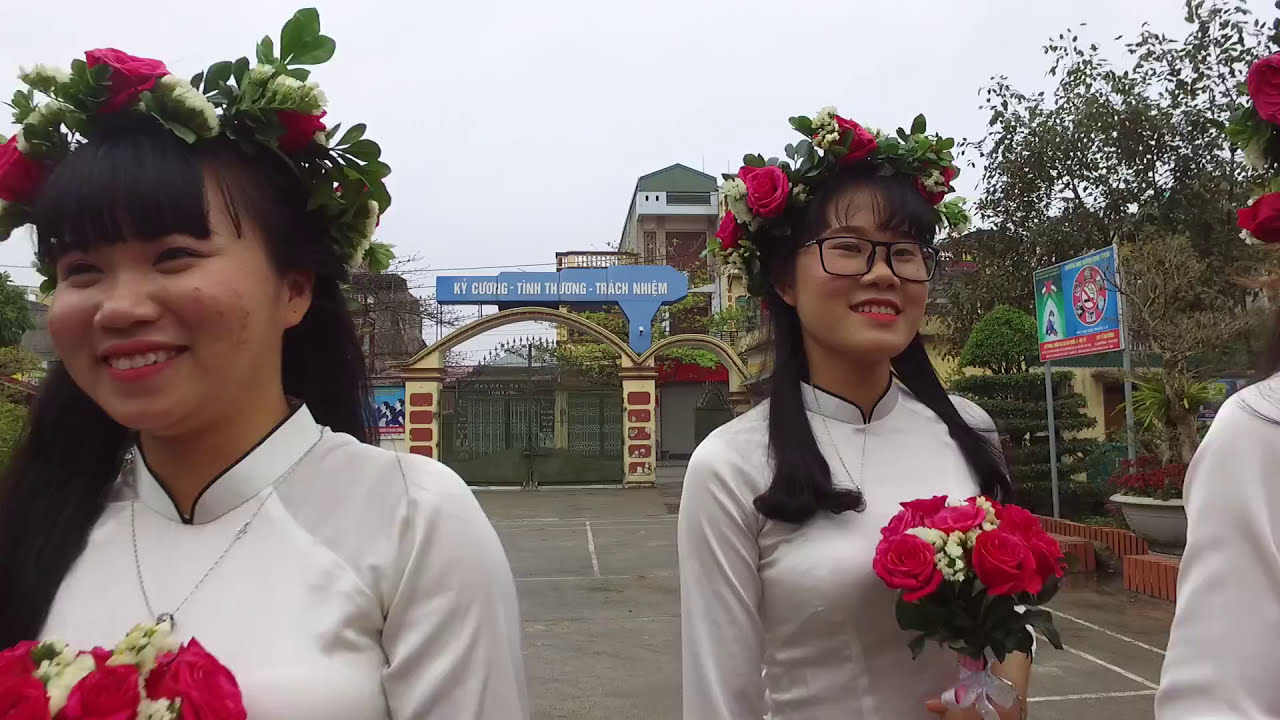This color photograph, oriented in landscape mode, features two smiling Asian women wearing traditional, silky white dresses with black-lined, stand-up collars. Both women have black hair with bangs and are adorned with silver necklaces. On their heads, they wear garlands of red roses interspersed with greenery, matching the bouquets they hold in their hands. The woman on the right is distinguishable by her black square-framed eyeglasses.

The setting appears to be an outdoor area, possibly a parking lot, bordered by a green gate and featuring some trees and brickwork. Overhead, there's a blue sign with white writing in a foreign language that cannot be read. The sky is overcast, adding a gray hue to the daylight scene. An arch structure and a tall building are also visible in the background, along with another sign in a foreign language and a partially visible person cropped off on the right side of the image.